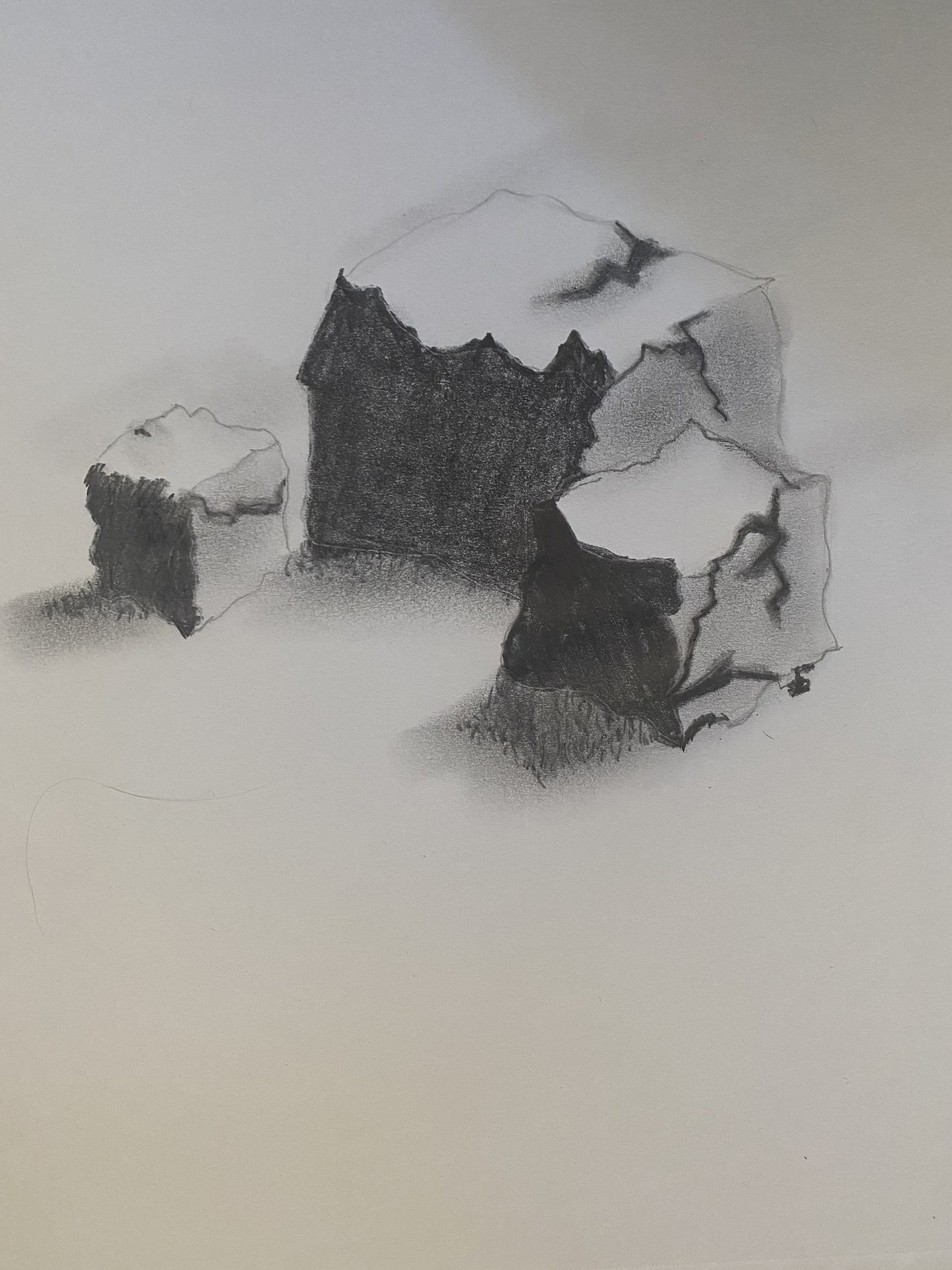On a stark white background, a charcoal sketch occupies the upper half of the page. This meticulously crafted drawing features three square objects of varying sizes, each enhanced with skillful shading primarily on their left sides and bottom left corners. The objects, strategically placed on a diagonal axis, reveal a fascinating interplay of light and shadow.

Starting from the left, the first object resembles a rugged piece of rock, its surface starkly white yet heavily shaded on its left panel. A prominent dark gray line carves through the right side of this cube, suggesting a significant crack or crevice.

In the center, the largest object dominates the composition. It too is shaded on the left side, with additional shadows cast toward the lower diagonal on the left. This cube displays two major cracks and a jagged top edge that intricately detail its weathered surface.

To the right, slightly further forward, lies the third and final object, distinguishable by its more rectangular shape. The shading here also targets the lower left corner, enhancing the texture and depth of the sketch. This rock is marked by two deep crack lines in dark gray, completing the visually compelling trio.

The artist's deft use of shading and line work breathes life into this composition, transforming simple sketches into evocative representations of rough, fractured rocks.